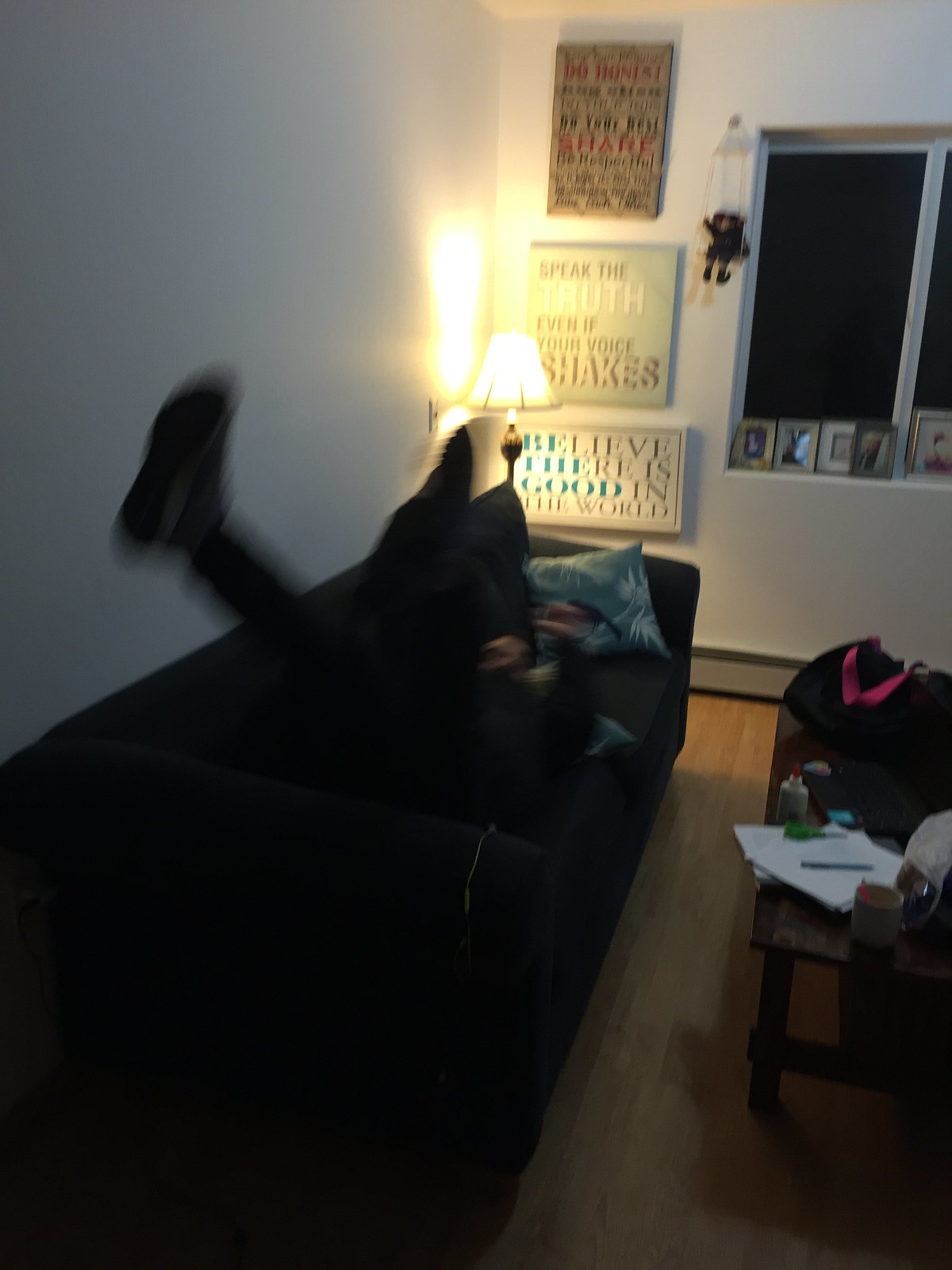In the image, a white wall spans the background with sections visible in the top left and top right corners. A couch sits against this wall, upon which a person is resting, their body reclined and one leg propped up. Behind the couch, several inspirational signs adorn the wall. One sign encourages, "Be honest, do your best," while another reads, "Speak the truth, even if your voice shakes," and yet another proclaims, "Believe there is good in the world."

To the left of the couch stands a lamp with a visible lampshade, casting its light and creating a shadow on the right side of the frame. Above the couch, several ropes hang down, indicating perhaps a decorative feature or part of window dressings.

A window with a darkened appearance is also present in the scene, edged by a windowsill that holds several framed photos. Below this, a wooden table is partially visible, cluttered with various papers, adding a touch of daily life and activity to the setting.